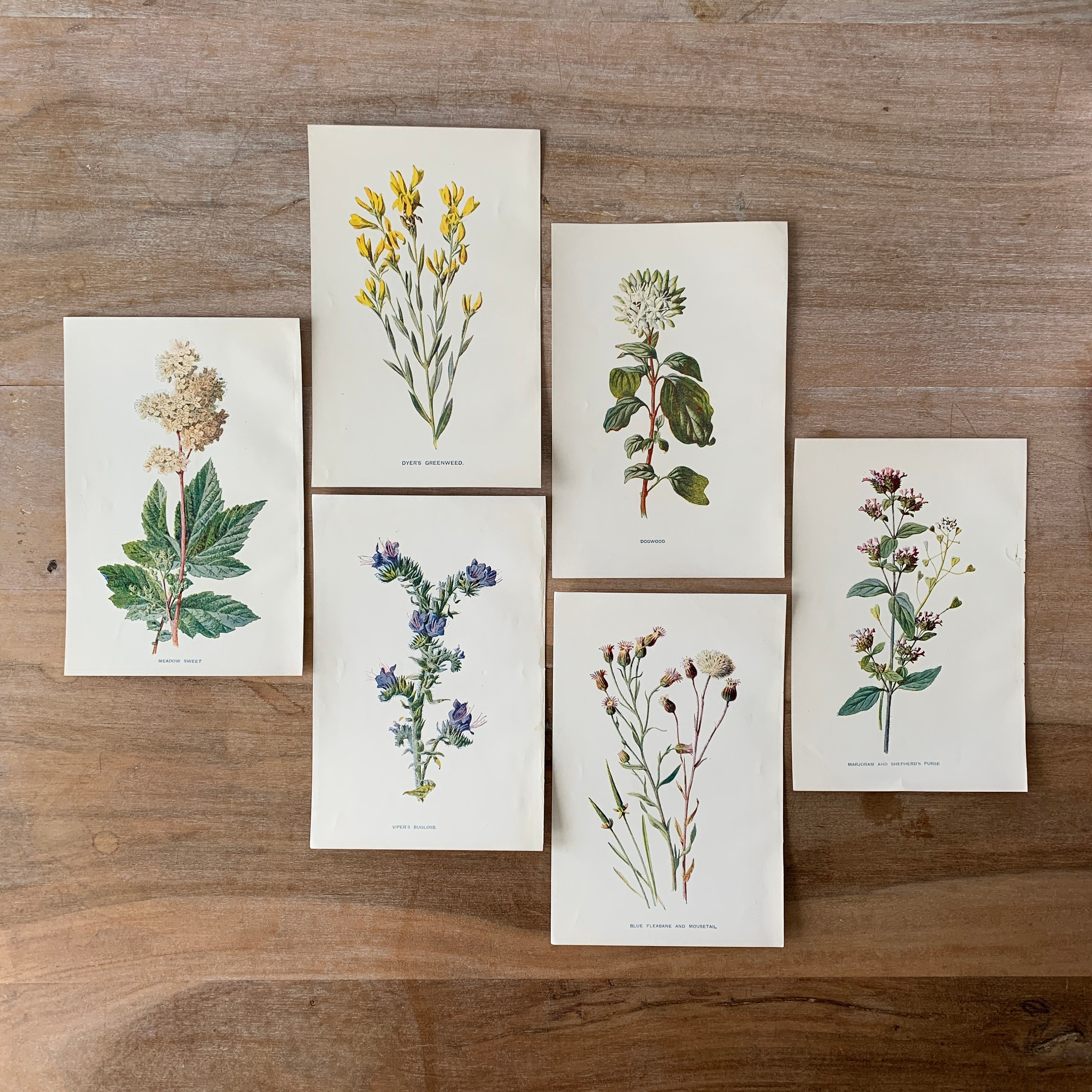The image contains six vertical white cards laid out on a wooden surface that transitions from a lighter color at the top to a darker shade at the bottom. Each card features a detailed drawing of a different type of flower with accompanying small black text, likely denoting the flower names, though the text is too tiny to read. Starting from the left, the first card showcases a flower with white petals and green leaves. To its right, the second card depicts a flower with small yellow blossoms, and the third card displays a plant with larger purple flowers. Adjacent to these, the fourth card features what appears to be a dandelion. The fifth card includes smaller purple flowers, and the sixth, positioned on the far right, also illustrates purple flowers. The cards are arranged in a visually appealing pattern: one card on the far left, a stacked pair of cards slightly to its right, another pair positioned lower down, and the final single card further right, creating a balanced display of botanical illustrations against the variegated wooden backdrop.